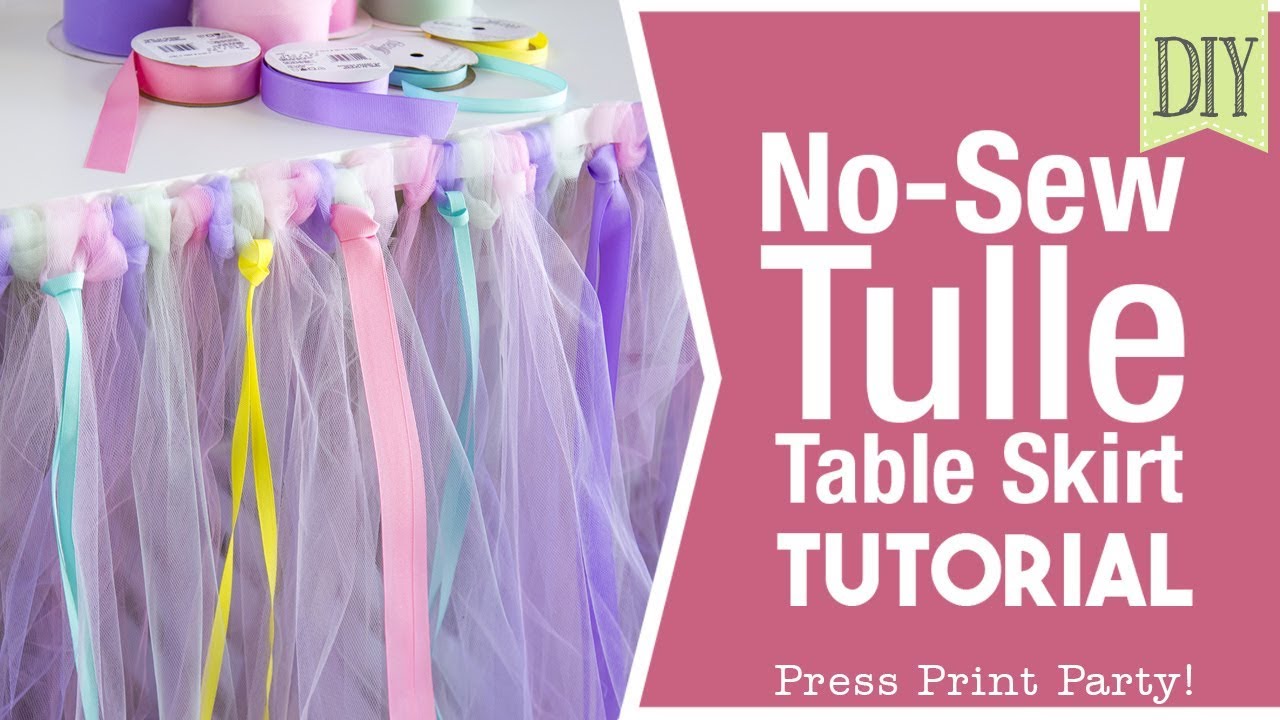The poster image features a promotional piece divided into two sections. On the left side, a photograph displays a white tabletop adorned with pastel-colored tulle and ribbons—available in shades of blue, yellow, pink, and lilac—some of which are slip-knotted around the table edge. In addition, spools of ribbon are neatly arranged in a circular manner on the tabletop. To the right, set against a rosy mauve background, white text prominently reads, "No Sew Tulle Table Skirt Tutorial: Press Print Party." A green bookmark symbol in the top right corner, shaped with a negative V cut at the bottom, bears the word "DIY" in black. This visually appealing composition aims to promote a DIY table skirt tutorial, ideal for creating decorative table settings for parties.